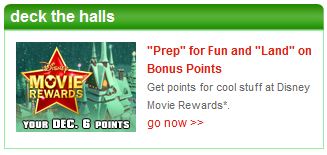The image appears to be a promotional graphic for Disney Movie Rewards, a rather dated service. The design of the image reflects its age and era. At the top, there is a green banner with white text that reads "deck the halls" in all lowercase lettering. The entire image is framed by a green border. 

On the left side, there is a small inset image featuring the Disney Movie Rewards logo, which consists of a gold-edged star with a red fill. Adjacent to the logo, the text mentions "Your December 6th points." The background behind this inset includes a cityscape or castle with snow-covered roofs, adding a festive touch.

To the right side of the image, the background is white with red text at the top that says "prep" in quotation marks and "land" also in quotation marks, suggesting fun and bonus points. Below this header, black text reads, "Get points for cool stuff at Disney Movie Rewards," followed by an asterisk. Beneath this, the phrase "go now" is written in all lowercase red text, accompanied by two red arrows pointing to the right, indicating a call to action.

Given the overall design and context, it is likely that this image was once part of a webpage promoting Disney Movie Rewards during a holiday season.